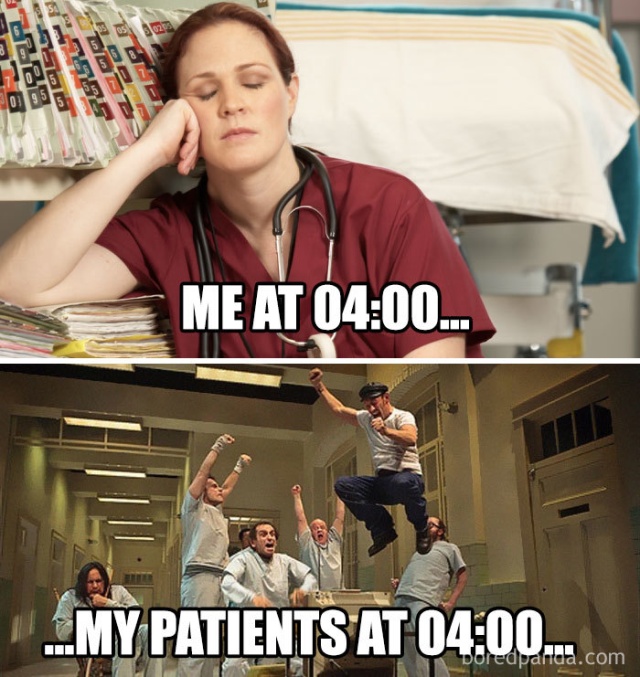The image features a meme format divided into two sections. The top half shows a female medical professional, dressed in scrubs with a stethoscope around her neck. She appears exhausted, leaning on her hand with her eyes closed, as if taking a brief nap. The setting suggests a hospital environment, indicated by patient files and a covered bed in the background. The caption on this image reads, "me at 4:00."

In contrast, the bottom half depicts a lively scene of seven individuals, most of whom are dressed in hospital scrubs, with one person in blue jeans and a T-shirt. They are energetically jumping, singing, and holding hands, with their mouths open in joyful expression. This image is accompanied by the caption, "my patients at 4:00."